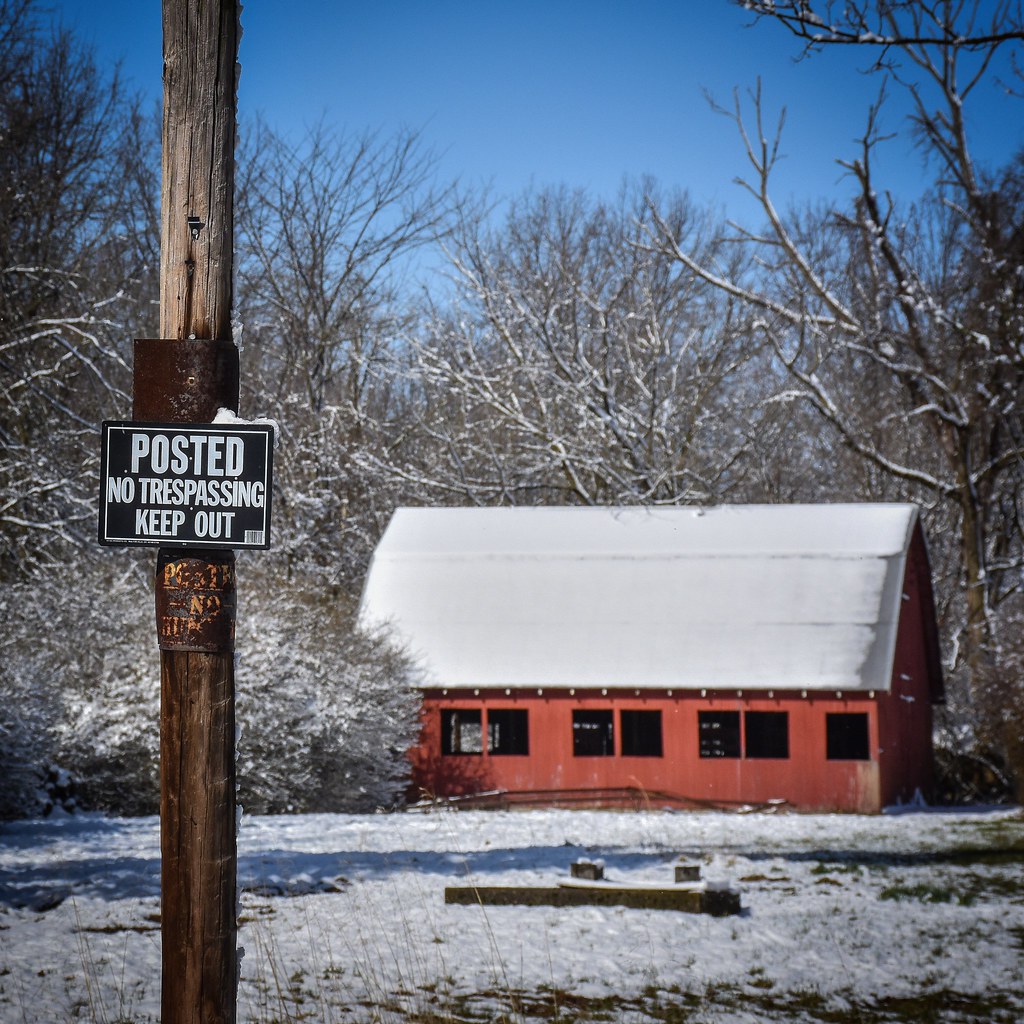The image depicts an old, somewhat dilapidated red barn nestled amidst a snow-covered winter landscape. The barn’s wooden exterior, painted a faded red with patches of peeling paint, contrasts sharply with the pristine white snow that blankets its steeply angled roof and the ground below. Dark, open windows hint at an abandoned interior. Surrounding the barn are snow-laden deciduous trees, barren of leaves, and to the right, an evergreen tree. A worn wooden post with a black and white sign reading "POSTED, NO TRESPASSING, KEEP OUT" stands prominently in the foreground. Additional details reveal a scattering of green grass peeking through the snow and a set of short posts on the ground, possibly marking an old parking area. The sky above is a clear, bright blue, adding a touch of serenity to the stark winter scene.